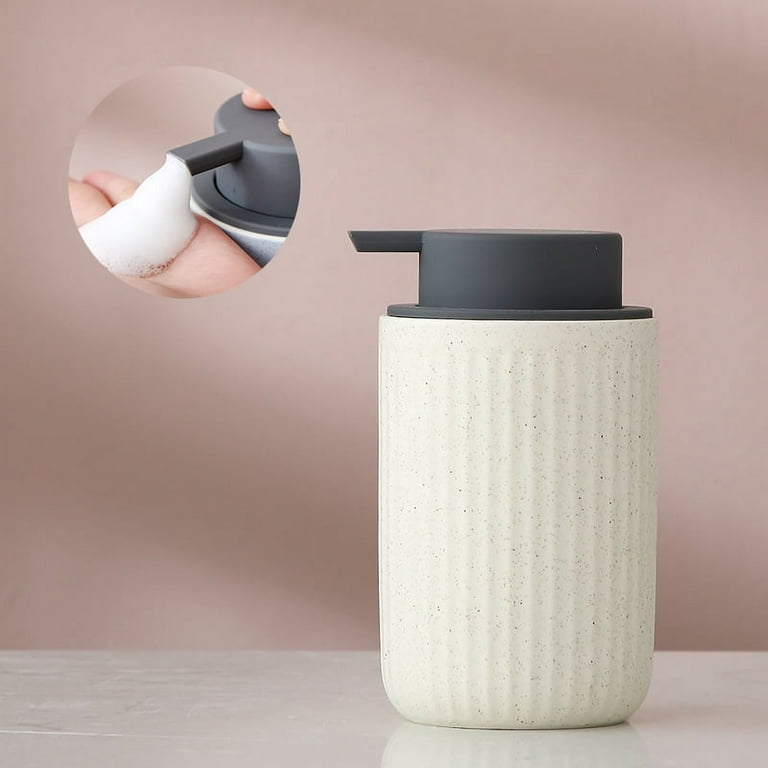The image is a detailed advertisement for a foaming soap dispenser. The background features a rose-pink or mauve color, lending a soft and clean atmosphere to the shot. The dispenser, which takes on a cylindrical, cup-like shape, is predominantly white with subtle gray speckles, mimicking a stone-like texture, and sits on a small segment of a white marble-like table at the bottom of the image. The top of the dispenser is equipped with a pump-style mechanism in a grayish-brown hue. Notably, in the upper left-hand corner of the photo, there's a circular inset displaying a close-up demonstration. This inset shows a person pressing the pump to dispense white foamy soap into their flat, open hand. The clarity and brightness of the image, alongside the blurred background, emphasize the crisp, clean experience of using the soap dispenser.